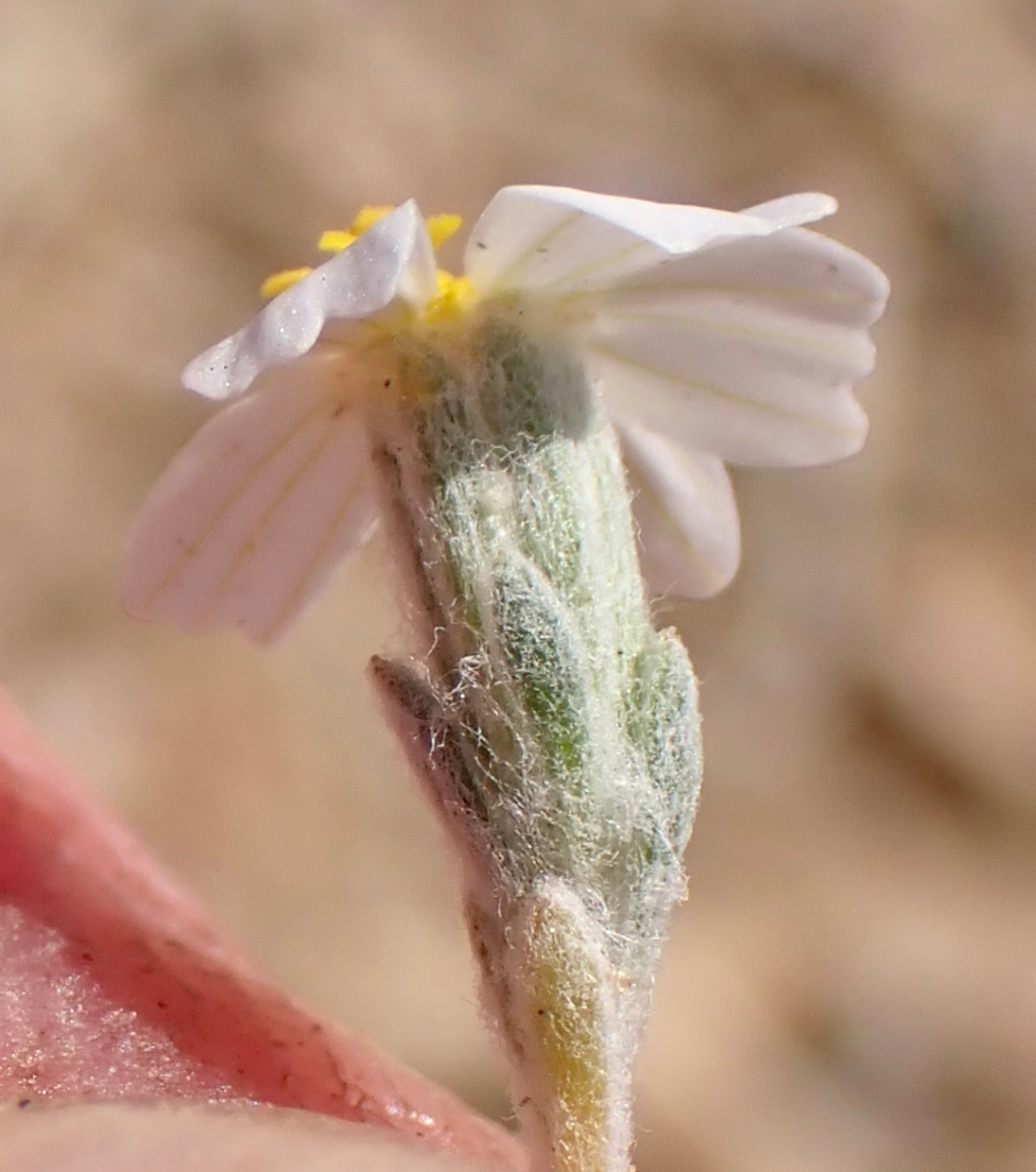This close-up photograph captures a singular white flower with delicate petals that radiate outward, emphasizing its sunny and serene setting. The center of the flower is adorned with a yellow, slightly fluffy, and protruding core, reminiscent of a dandelion. The background is blurred into a light brown or beige hue, suggesting an outdoor environment basked in sunlight, predominantly streaming in from the right side of the image. The green stem of the flower appears to be enveloped in a thick, white, fuzzy material—evocative of spiderwebs or cobwebs—that stretches from just below the petals down to the leaves. Additionally, a pink, fleshy texture is visible near the flower, adding a subtle contrast to the light, airy aesthetic of the image.